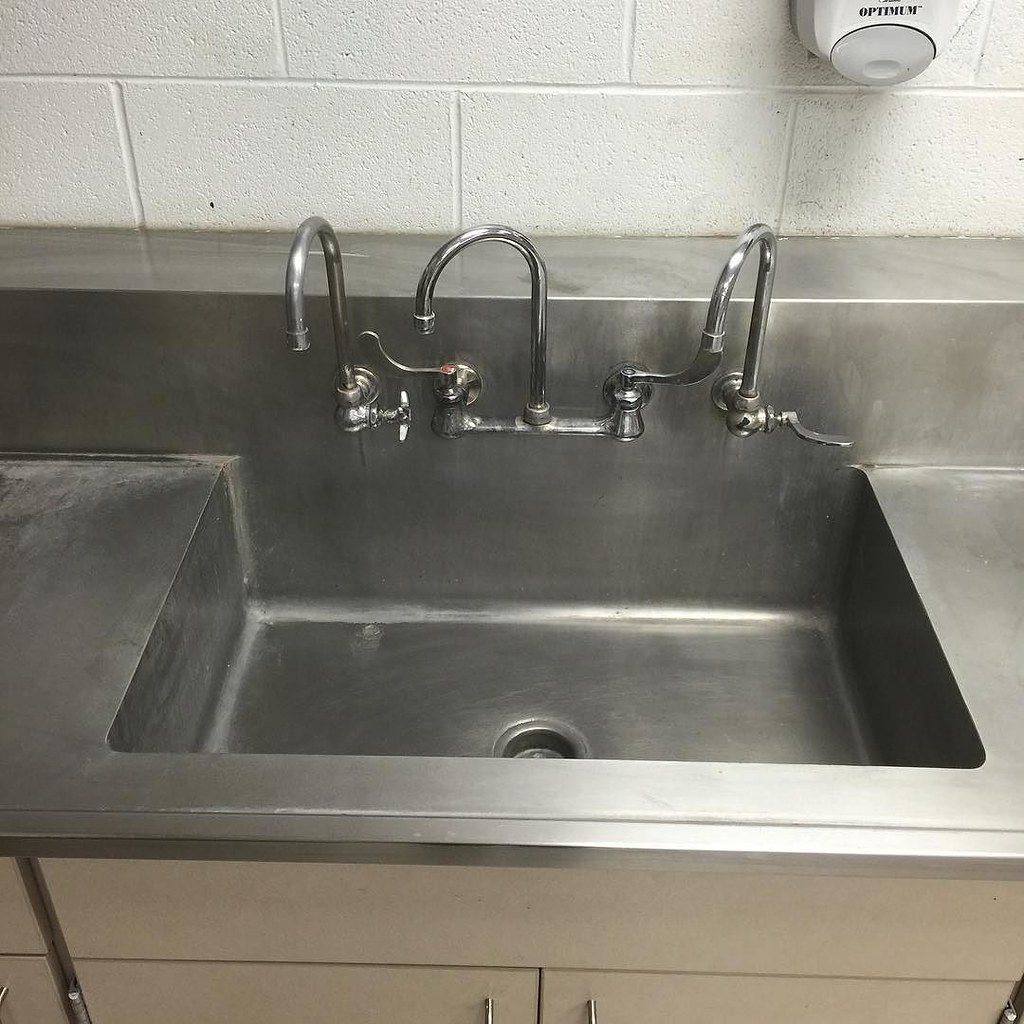This photograph features a large rectangular stainless steel sink with one deep basin and three faucets: a central faucet with separate hot and cold handles, flanked by a faucet on each side, each with a single dial. The sink is integrated into a stainless steel countertop and backsplash, creating a sleek and uniform appearance. Below the sink are tan cabinets with black specks and stainless steel handles. The wall behind the sink is made of painted white cinder blocks. Mounted to the top right of the sink area is a white plastic soap dispenser with a gray lever that reads "Optimum."